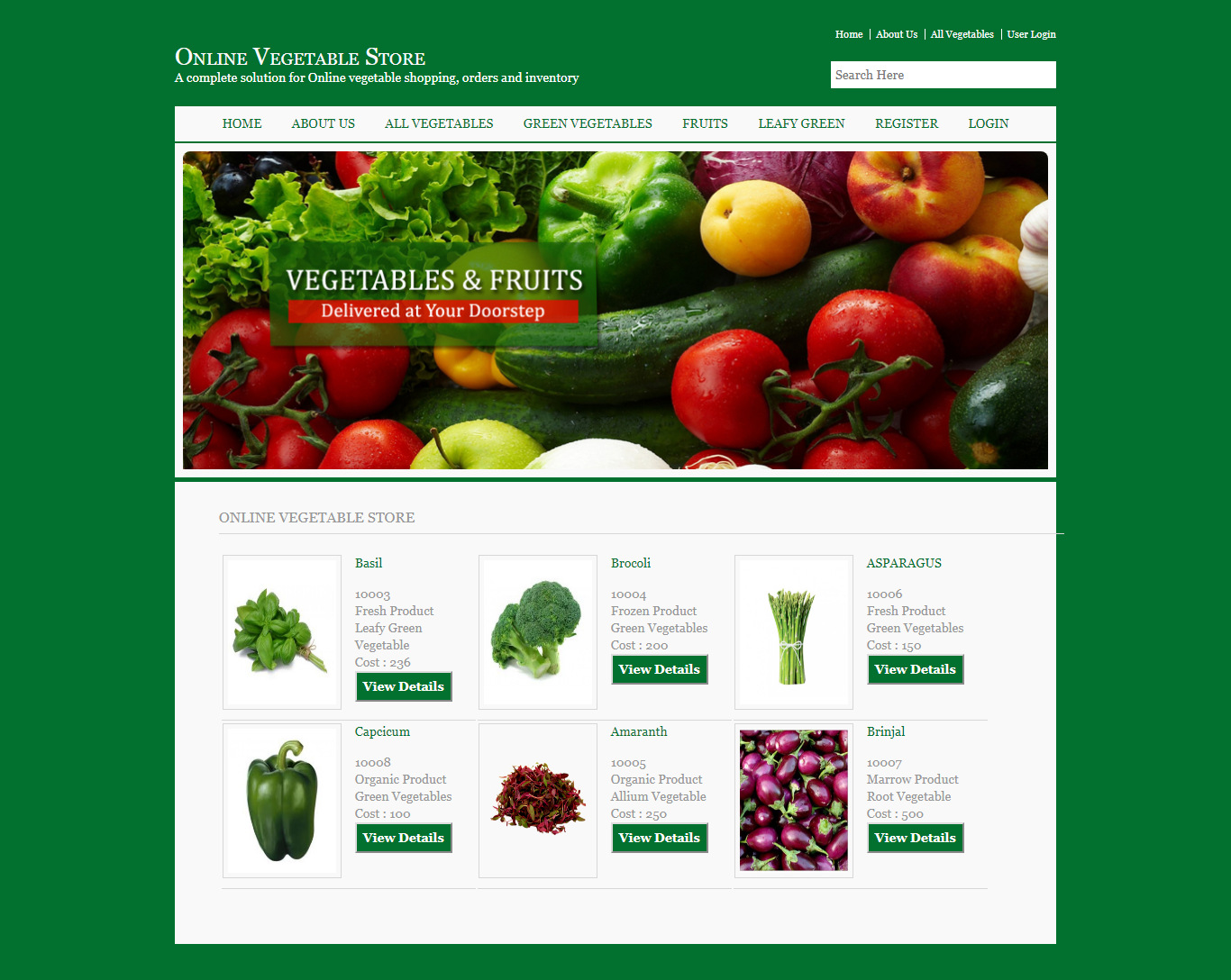This screenshot features a vibrant green background, with a prominent white square centered slightly offset towards the bottom. At the top left, the text "Online Vegetable Store" is displayed in white, accompanied by a smaller line of text just beneath. To the top right, a white search bar is flanked by a horizontal list of menu items: "Home," "About Us," "All Vegetables," and "Login."

Beneath this, within the white square, another row of navigational options appears at the top: "Home," "About Us," "All Vegetables," "Green Vegetables," "Fruits," "Leafy Greens," "Register," and "Login."

Centrally featured within the white square is a rectangular image showcasing fresh produce, including tomatoes, green apples, peaches, green lettuce, and a cucumber. Adjacent to the image, a vertically positioned green rectangle centered from top to bottom displays the words "Vegetables and Fruits" in white. Below this, a red horizontal rectangle reads "Delivered at your doorstep" in white text.

The bottom section of the white area is divided into vertical rectangles, arranged in six columns and two visible rows. The top of this section is labeled "Online Vegetable Store" in gray text. Each vertical rectangle showcases an image of a vegetable, such as basil, with descriptive text to the right and a green "View Details" button. Additional vegetables displayed include broccoli, asparagus, green peppers, and radishes.